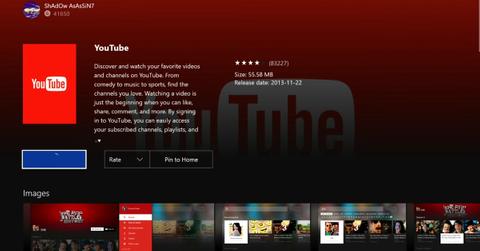The image displays a YouTube interface with a distinct color gradient background—dark at the bottom and red at the top. The YouTube logo is subtly visible behind the content. On the left side of the screen, a red rectangle prominently features the YouTube logo. Adjacent to this, the word "YouTube" appears in white letters, and beneath it is additional white text, followed by a series of four stars.

Continuing to the right, the screen shows pricing information with more white text underneath. Midway through the left side, a blue rectangle is visible, and adjacent to this is a rate icon. Next to the rate icon, there is a text suggesting a transition to the "home" section.

At the bottom left corner, the word "images" is displayed in white letters. Below this, a series of movie titles is arranged horizontally, with five titles spanning from left to right. One of the movie titles stands out with a red top and black bottom and features a red drop-down menu icon. Successively to the right are three blurred-out movie screens. The sequence concludes with another movie title, also characterized by a red top and black bottom.